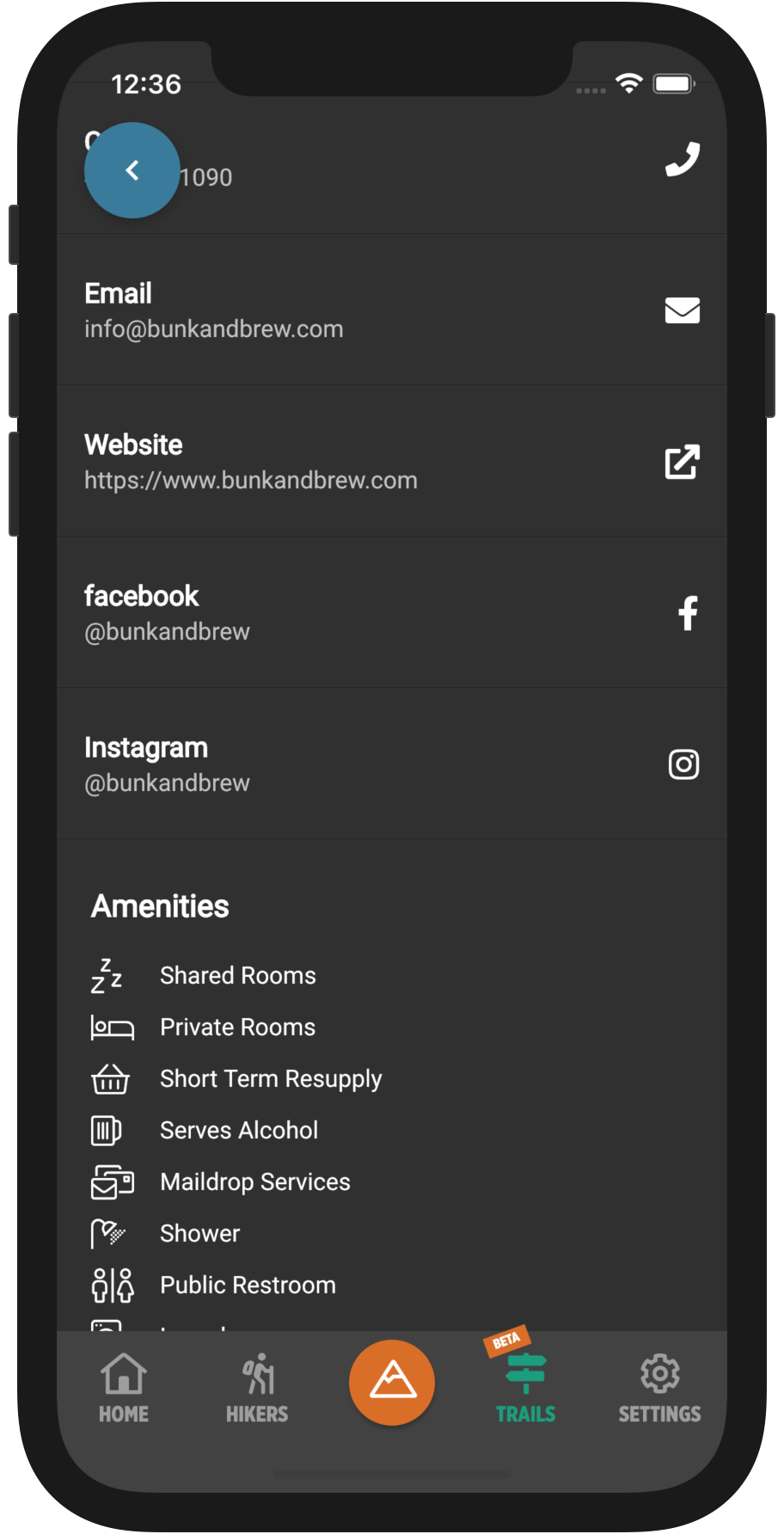This is a detailed digital illustration of a smartphone display, emphasizing the screen's content. The phone's exterior, which is entirely black, prominently features the power button as well as volume control buttons—three on the left and one on the right, subtly protruding from the casing.

The screen itself shows the time in the upper left corner—12:36 in white print. The status bar also indicates a fully charged battery and active Wi-Fi connection. Following down the right side, we see icons for a phone, email (represented by an envelope), upload (an arrow symbol), Facebook (an "F"), and Instagram (a camera icon). These icons correspond to various apps and functions.

Within the email section, the email address displayed is "info@bunkandbrew.com." The website section presents the URL "https://bunkandbrew.com." Both Facebook and Instagram handles are "@bunkandbrew."

Towards the bottom, a section titled "Amenities" features various icons, each paired with descriptions, listing the available amenities in a detailed manner. This meticulous layout ensures users can easily find and access the needed information.